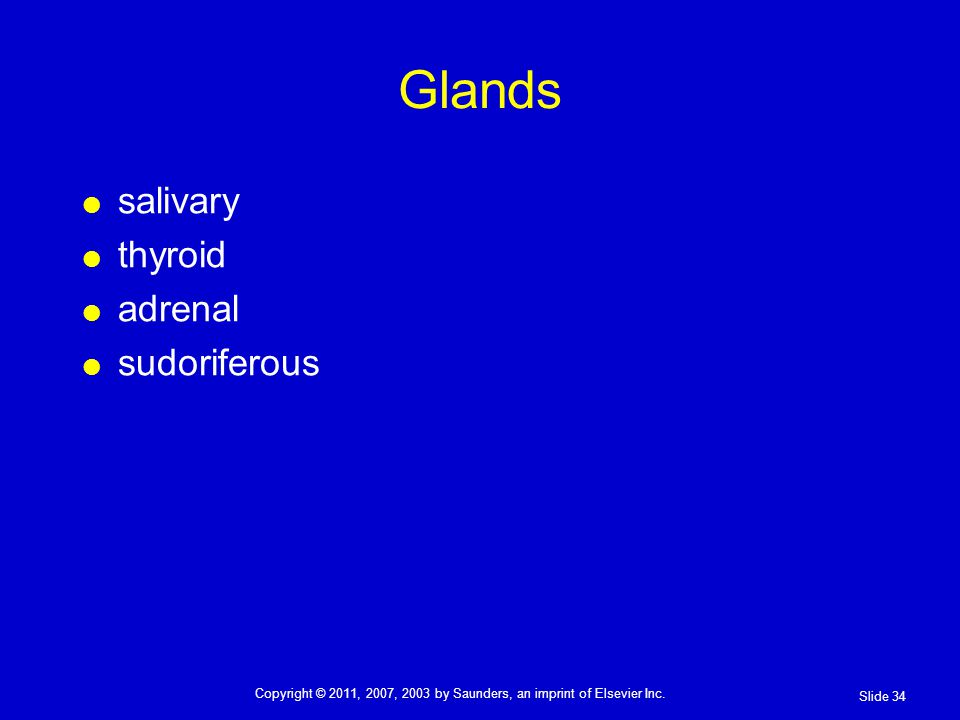The image is a PowerPoint training slide, likely intended for a class or medical school. It features a solid bright blue background with no gradient, making it look quite plain and uninteresting. At the top center, the title "GLANDS" is prominently displayed in yellow text. Below the title, aligned to the left, is a vertical list of four points each marked by a yellow dot. The bullet points list the following glands in white text: "Salivary," "Thyroid," "Adrenal," and "Sudoriferous." At the bottom center of the slide, it states "© 2011, 2007, 2003 by Saunders, an imprint of Elsevier Inc." In the bottom right-hand corner, the slide number "34" is displayed.